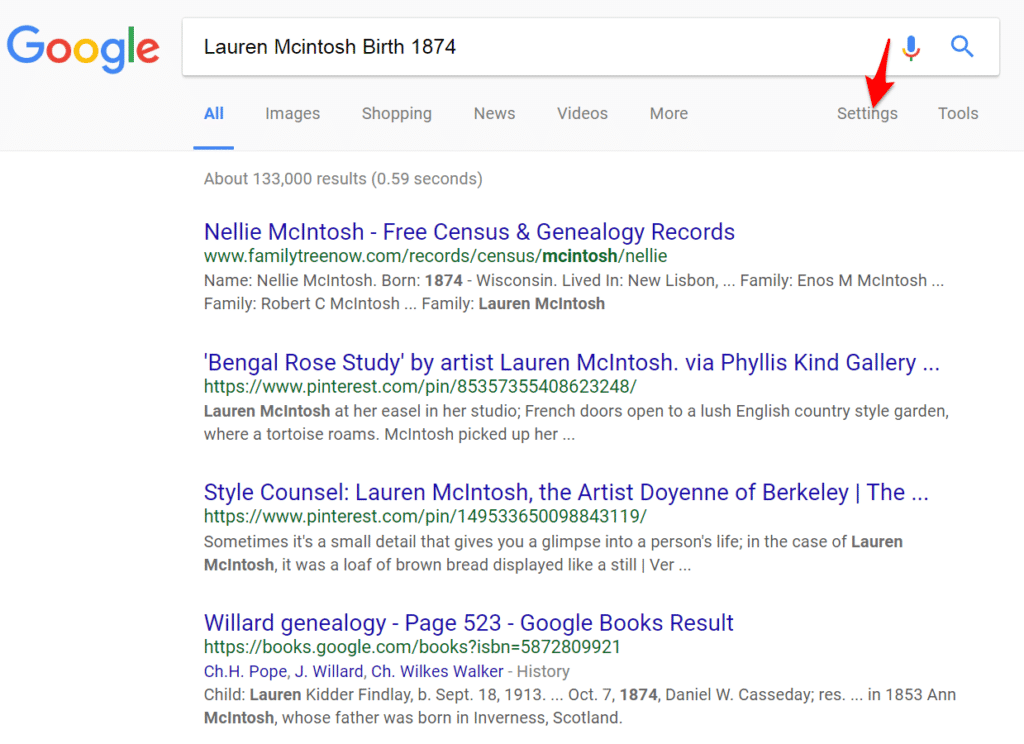This is a screenshot of a Google search home page. The search bar shows the query "Lauren McIntosh birth 1874." There is a red arrow pointing at the word "Settings" located at the top right of the page. The navigation options available at the top include All, Images, Shopping, News, Videos, More, Settings, and Tools. The search engine has produced approximately 133,000 results in 0.59 seconds.

The first search result prominently displays "Nellie McIntosh - Free Census and Genealogy Records" from www.familytreenow.com. This entry mentions Nellie McIntosh, born in 1874 in Wisconsin, who lived in New Lisbon. The record also lists family members including Enos M. McIntosh, Robert C. McIntosh, and Lauren McIntosh, who is the subject of the search.

The second result references "Bingle Rose Study" by artist Lauren McIntosh via Phyllis Kind Gallery, with a link to Pinterest, showing Lauren McIntosh at her easel in her studio.

The third result is titled "Style Council: Lauren McIntosh, The Artist of Berkeley," also linked to Pinterest.

Additional results include a page from "Willard Genealogy" available on Google Books, featuring Lauren Kidder Finley and other entries that match the birth year 1874 for individuals with the last name McIntosh.